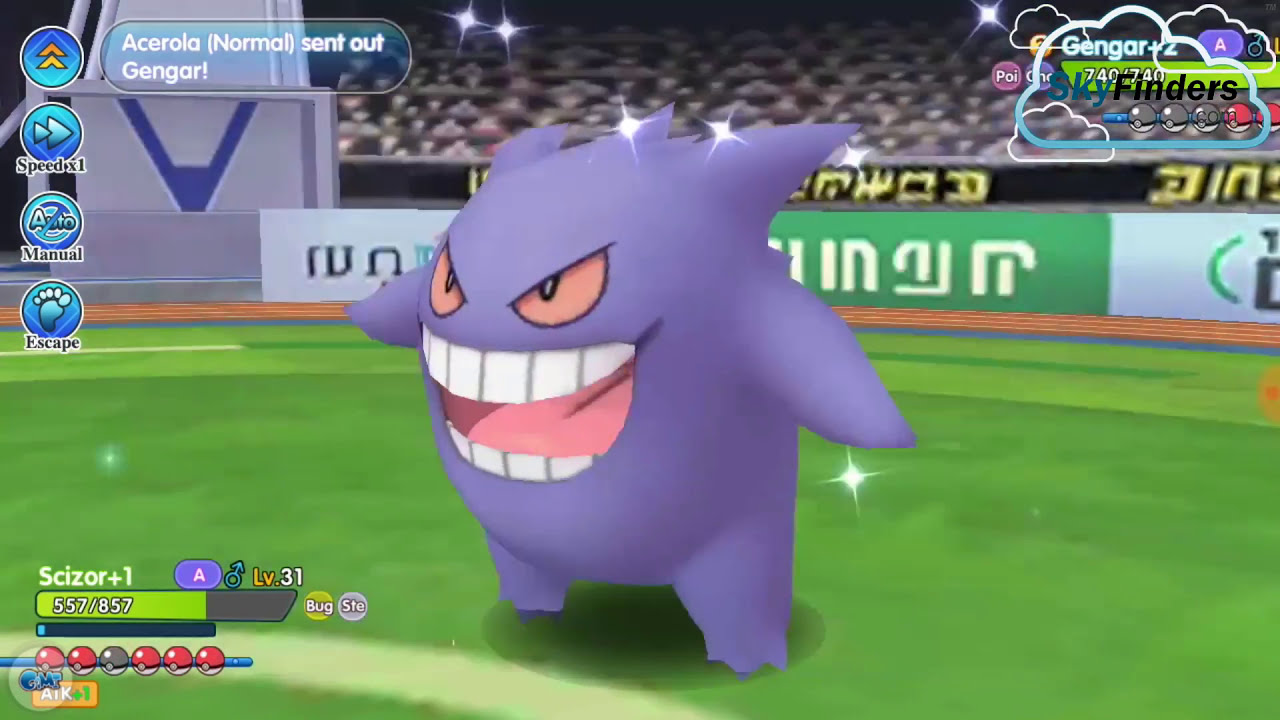The image is a screenshot from a Pokemon-themed fighting video game, featuring a central character, Gengar. Gengar is depicted as a ghost-like creature with light purple, spiky skin, a round body, and large, slanted pink eyes giving it a somewhat sinister appearance. It has a wide-open mouth, showcasing two rows of flat, white teeth, a large pink tongue, and a pink mouth interior. The scene takes place on a green, pixelated surface resembling a grassy field within a stadium. In the top left corner, it reads "Acerola Normal Sent-Out Gengar," accompanied by various blue icons, including arrows pointing upwards and to the right. Additional game indicators such as health points and level information (Gengar at level 31 with 557 out of 857 HP) are present, indicative of an ongoing battle. The stadium background and the graphical style suggest a pixelated, classic video game aesthetic.